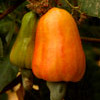The image features a close-up of a small, orange pepper prominently centered within a dark background. The pepper has an oblong shape with one end wider than the other, much like an upside-down bell pepper. A green stem is visible at the top of the orange pepper. To the left, partially obscured, is another pepper that is green but appears to be transitioning to an orange hue in some areas. This green pepper is only partially visible, with about a third of it in view. Both peppers occupy the central focus of the image, while the background remains dark, accentuating the vibrant colors of the peppers.